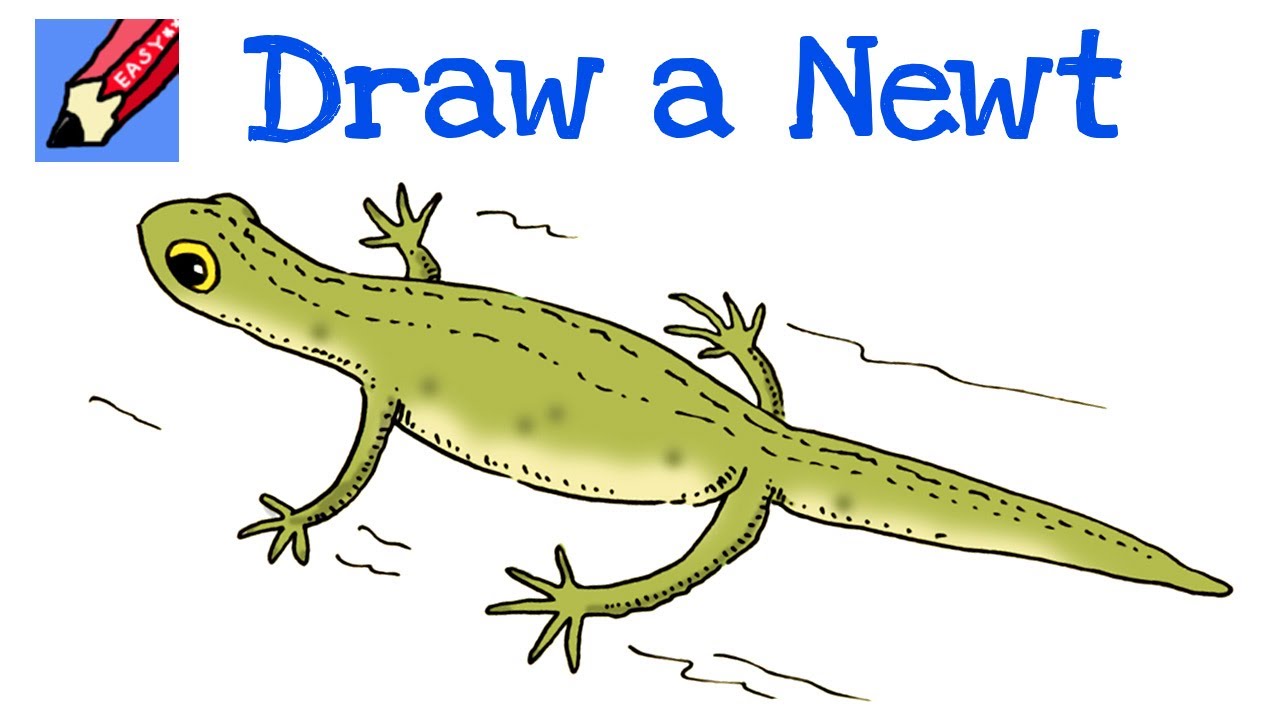The image is a detailed, cartoon-style drawing tutorial labeled "Draw a Newt" in blue text at the top. To the left of the text is a red pencil illustration within a blue box, inscribed with the word "easy." The newt itself is the focal point of the image, depicted in a walking pose with its head to the left. It is primarily green with a yellow underside and distinct green dots running down its back. Its eyes are large and yellow with black pupils. The front legs of the newt have four claws each, while the back legs have five claws each. The newt is shown fully, with four outstretched legs, a detailed body, and a long, straight tail. The entire scene is set against a white background, emphasizing the step-by-step drawing instructions.